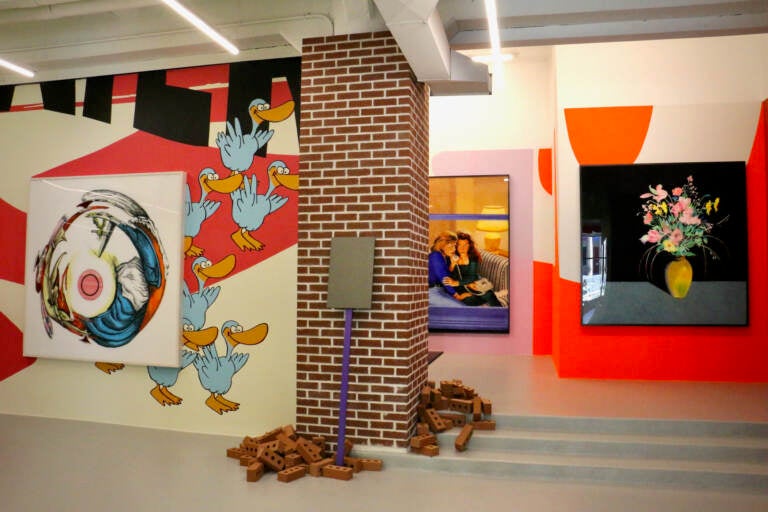The photograph depicts an art gallery showcasing a variety of artwork and artistic elements. On the left side, there's an abstract painting featuring a red circle at its center, with colors such as blue, white, yellow, orange, and red swirling around it. This painting is set against a mural of cartoon ducks, blue with yellow bills, walking in a line. Adjacent to this scene, a brick pillar stands, which has several bricks placed at its base, possibly as part of an installation. A blank gray sign on a purple pole is situated to the right of the pillar.

In the center background, a realistic painting captures two teenage girls from the 1980s, both on the phone and seated on a bed or couch. One girl is dressed in a blue long-sleeved shirt, while the other wears green. To the right, against a red, white, and orange wall, hangs a still-life painting of an orange vase with a yellow-green spot, filled with flowers in various colors—mainly pink, but also some yellow and shades of purple. The gallery is lit with harsh office lighting and features a short set of three stairs leading to the back section.